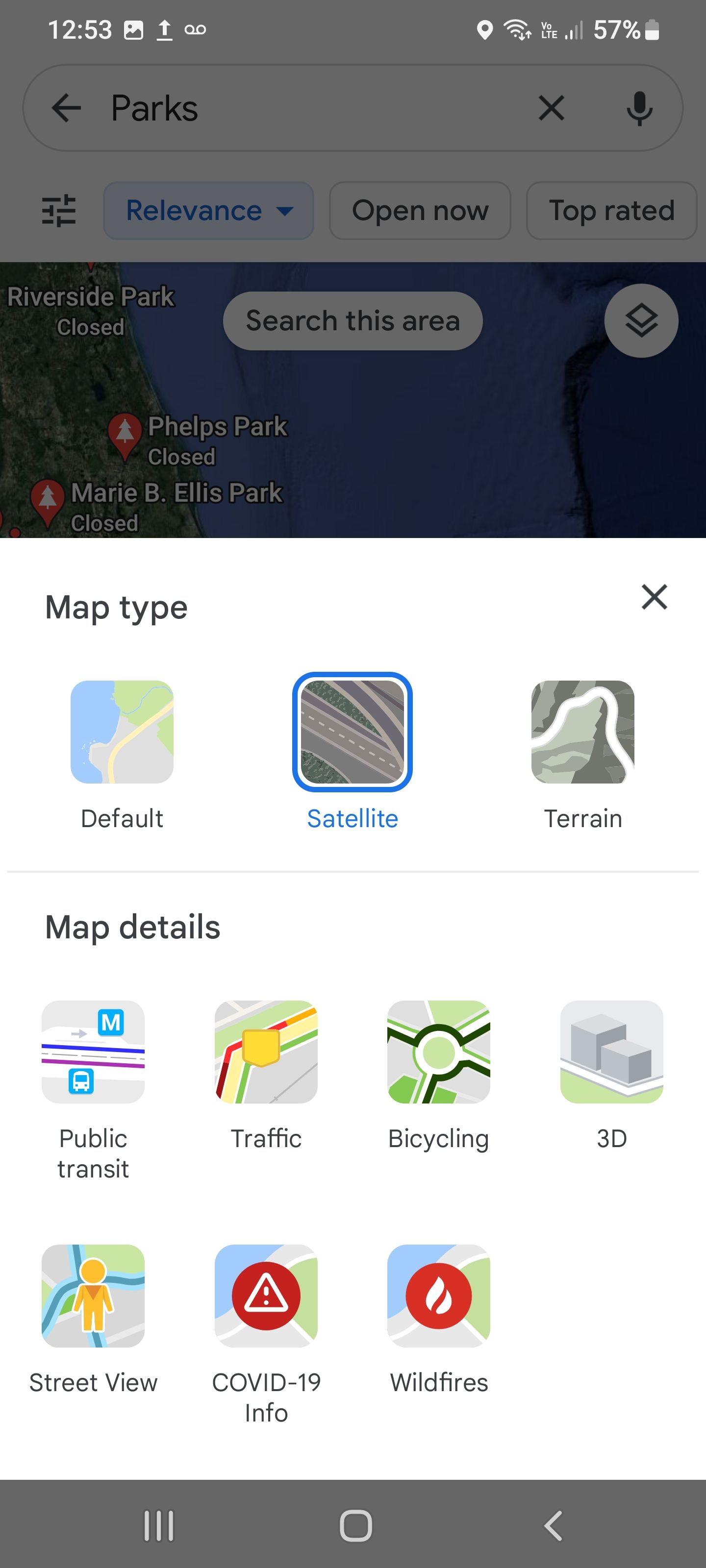This image, captured on a cellphone, features a search interface for parks. At the top, "parks" is typed into the search bar. Below the search bar are filter options labeled "Relevance," "Open Now," and "Top Rated," with "Relevance" selected. A button below this filter reads "Search this area." The search results show Riverside Park, Phelps Park, and Marie B. Ellis Park, all marked as "Closed."

The map display settings indicate that the current view is set to "Satellite," rather than "Default" or "Terrain." Map details offer icons for various features: public transit, traffic, bicycling, 3D view, street view, COVID-19 info, and wildfire information. Specifically, the top row includes icons for public transport, traffic, bicycling, and 3D view, while the second row includes street view, COVID-19 info, and wildfires.

At the bottom of the screen, a dark gray rectangle houses three vertical lines beside each other, forming a square, and an arrow pointing left on the right side, possibly indicating navigation or additional menu options.